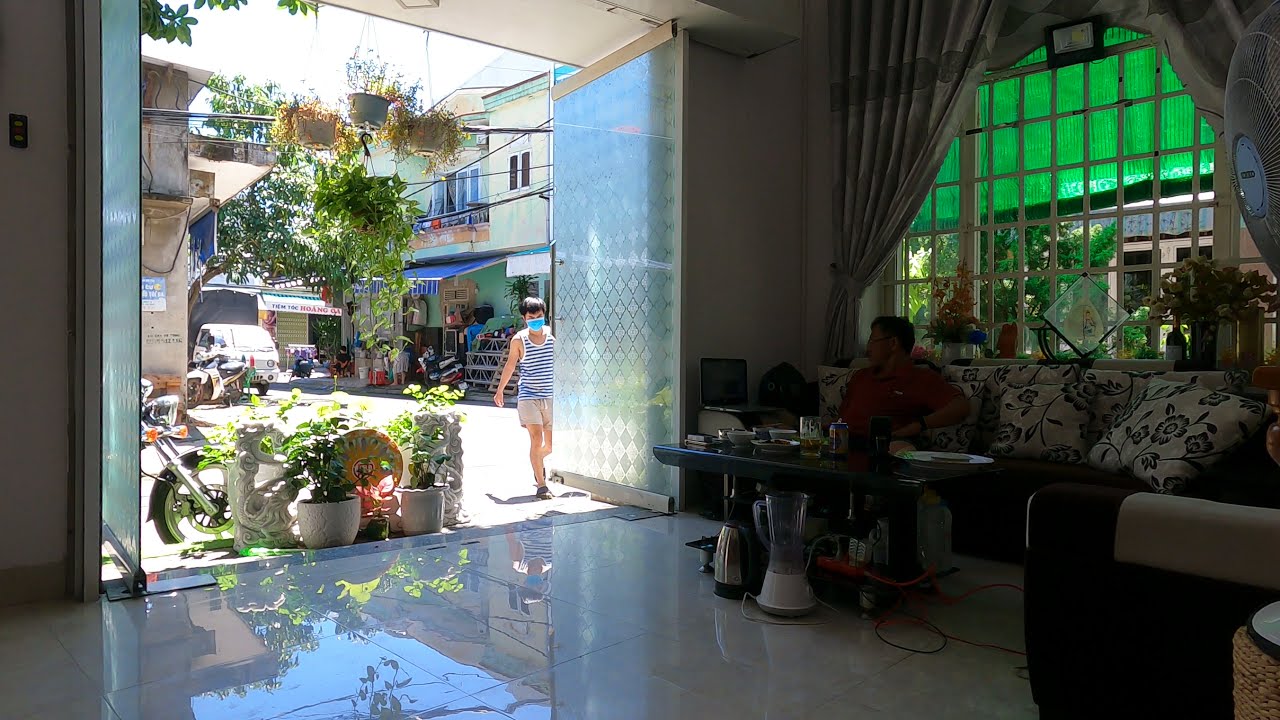The scene captures the interior of a living room-like space with a man seated on a brown couch accented by gray pillows featuring black floral designs. The couch, placed in the middle of the image, has a side table to the man's right, holding an open laptop computer. The floor is covered in reflective white tile. In front of the man is a rectangular coffee table, under which sit a blender, a kettle, and various bottles.

The room's large, glass doors with diamond patterns are opened outward, leading to a view of the street. Outside, by the doors, potted plants are visible, alongside the front end of a motorcycle. To the right, a man with short black hair, wearing a blue and white striped tank top, khaki shorts, and a blue and white face mask, is walking towards the camera.

In the street scene beyond, buildings with a mixture of white stone and brown areas stand, adorned with hanging plants and blue awnings. Some of these buildings appear to be older and possibly serve as apartments, completing the picturesque urban landscape.